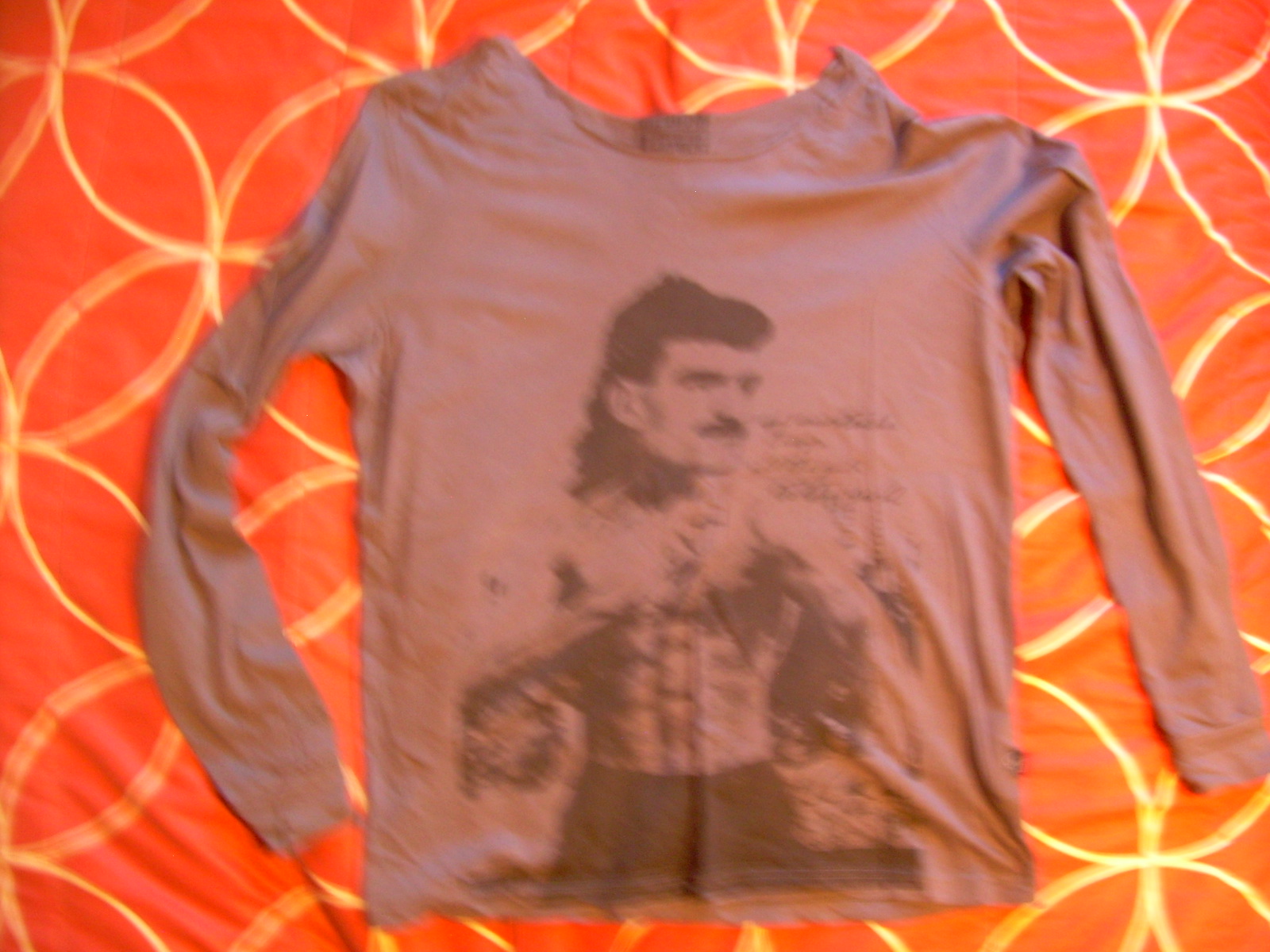This is a detailed photograph of a long-sleeved t-shirt, appearing to be mauve or reddish-brown in color, haphazardly laid out on an orange-red surface with a gold circular pattern. The shirt features a graphic print in black of a shirtless man with a mullet haircut and mustache, dressed in black pants and seemingly in a fighting stance with his arms raised to his chest. There is also script text next to the man's face, although it is unreadable due to blurriness. The shirt appears wrinkled and could be a youth-sized garment.